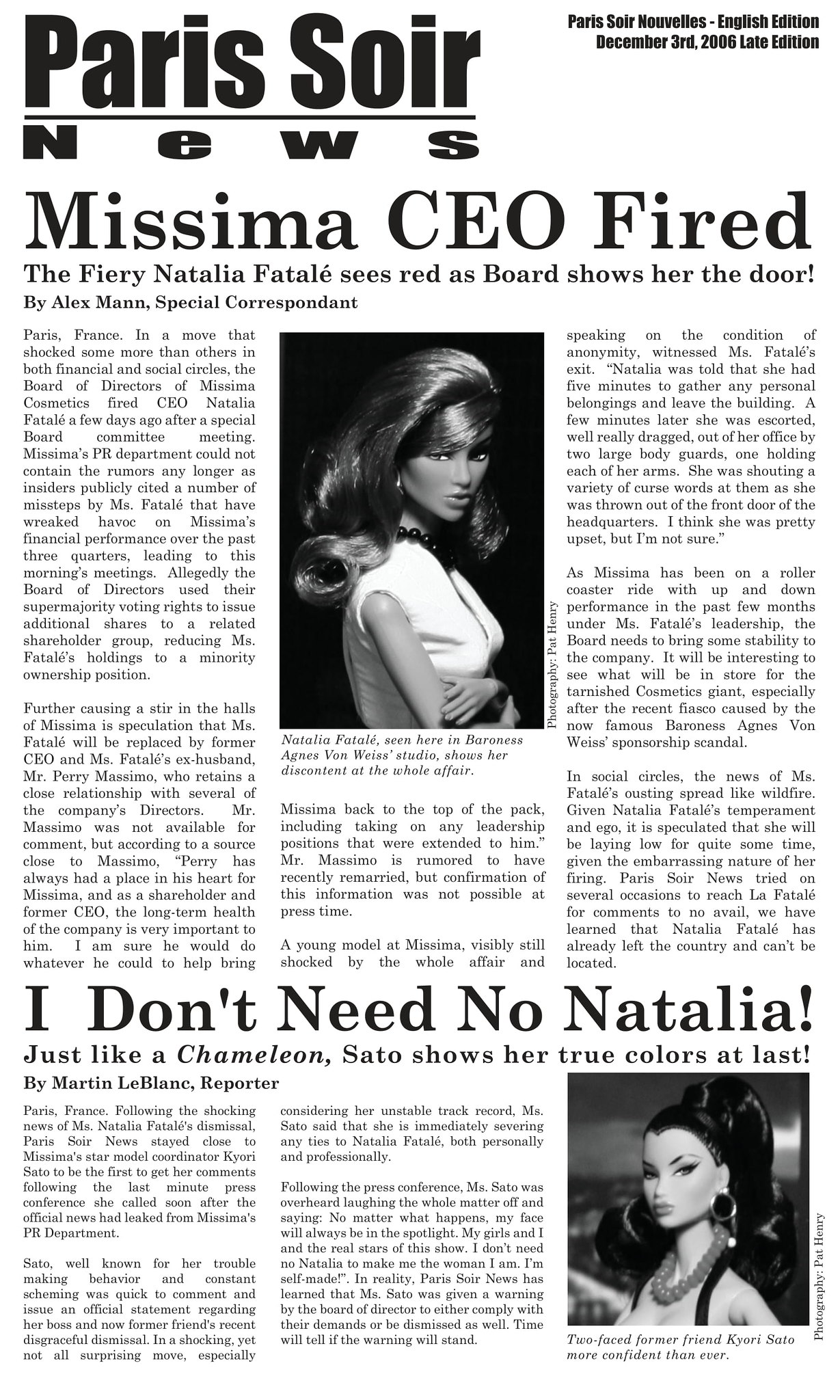This is a photograph of a newspaper-style page from "Paris Soir Nouvelles," English edition, dated December 3rd, 2006, late edition. The page features two main articles, both accompanied by black-and-white photographs of dolls. The top two-thirds of the page are devoted to the headline story: "Miss Sima CEO Fired." The subheadline reads, "The fiery Natalia Fatale sees red as the board shows her the door," with the article credited to special correspondent Alex Mann. The accompanying photograph depicts a doll with long blonde hair, arms crossed, identified as Natalia Fatale, shown in Baroness Agnes von Weiss's studio. Below this, another story appears under the headline, "I don't need no Natalia," with a subheadline, "Just like a chameleon, Sato shows her true colors at last." This article is also illustrated with a black-and-white photograph of a doll with black hair, situated to the right of the text. The entire background is white, and the text and images are in black and white, mimicking a traditional newspaper layout.